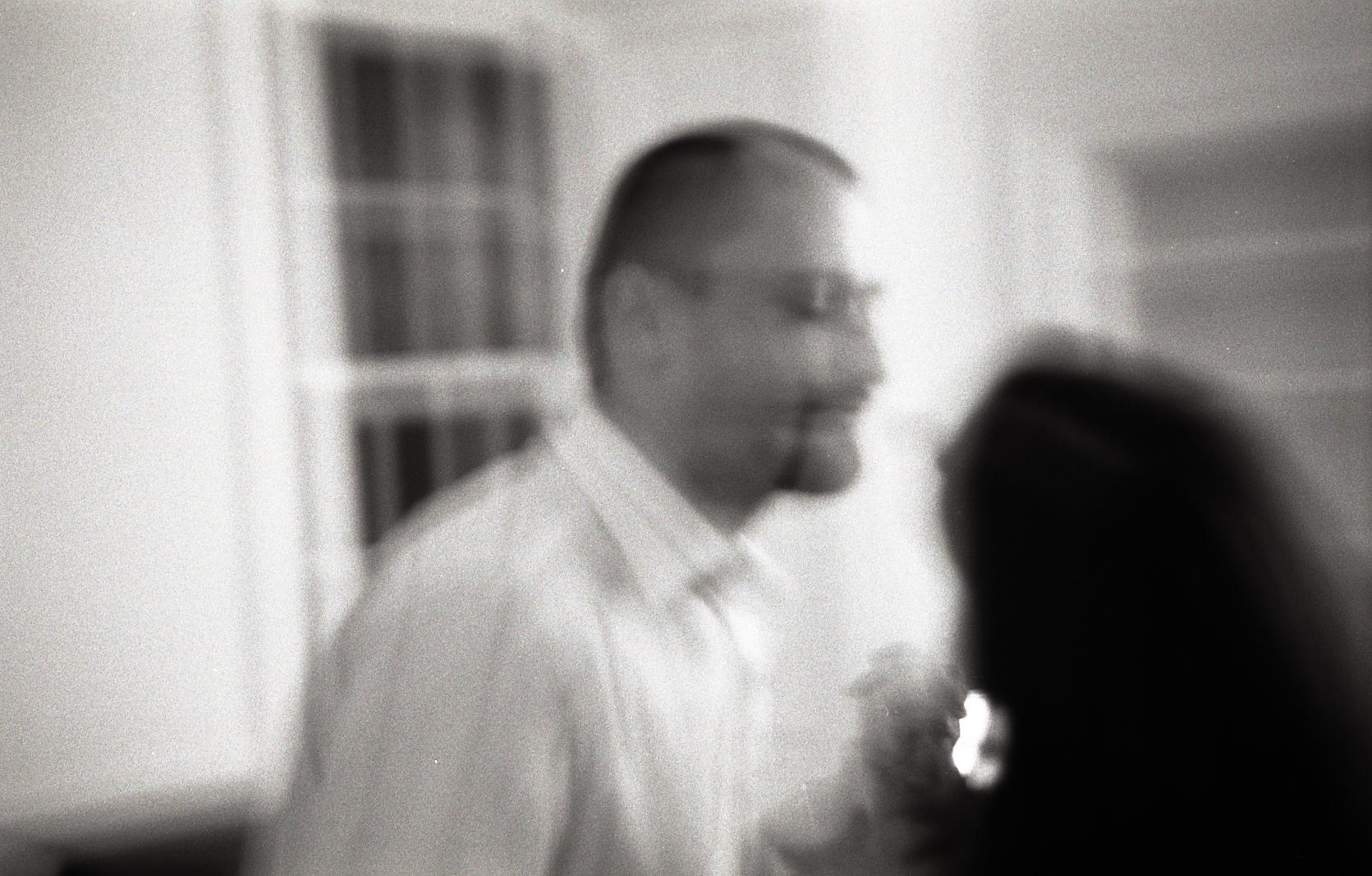In this blurry black and white photograph, the viewer is offered a close-up view of a man and a woman set against a sparse, monochromatic backdrop. The room's corner structure is delineated by two plain white walls, each featuring a window devoid of curtains, allowing the darkness of night to seep through. The focal point is the man's profile, characterized by his short-cropped hair and a distinctive facial hair pattern that includes a small mustache and neatly trimmed beard lines accentuating each side of his mouth. He wears a white dress shirt adorned with subtle stripes.

His eyes are closed and he leans slightly toward the woman, who stands just beside him, her long dark hair cascading and only her nose faintly visible in the dim light. A bright white reflective line runs between them, perhaps simplifying a moment of intimacy. The man's hand appears to be raised, fingers possibly clenched together, suggesting a gesture of affection or anticipation. They seem to be on the verge of sharing a kiss, captured in this poignant and evocative moment frozen in time.